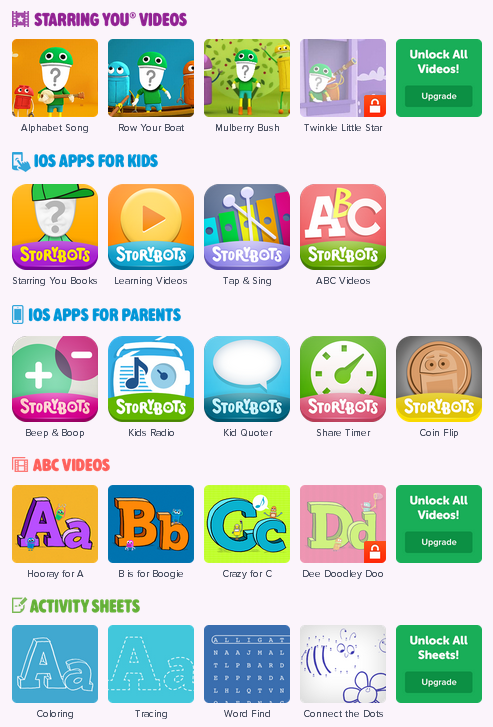Here's a cleaned-up and detailed caption for the image:

---

Screenshot of a video section on a children's app website or a children's app screen. At the top, a purple banner reads "Starring You Videos." Below, five video icons are displayed. The first four icons represent videos where children can insert their own faces for playback: "Alphabet Song," "Row Your Boat," "Mulberry Bush," and "Twinkle Twinkle Little Star," the latter of which features a lock icon in the bottom right corner, indicating it is locked. To the right of these videos, a green box prompts users to "Unlock All Videos - Upgrade."

Further down, a blue section titled "iOS Apps for Kids" presents four app thumbnails. Beneath that, a section labeled "iOS Apps for Parents" follows, showcasing five app thumbnails and titles. Next, an "ABC Videos" section appears, featuring five icons. The icon for the letter D is locked, and an "Unlock All Videos" thumbnail is positioned on the far right. Lastly, the "Activity Sheets" section includes five icons, accompanied by an "Unlock All Sheets" thumbnail on the far right.